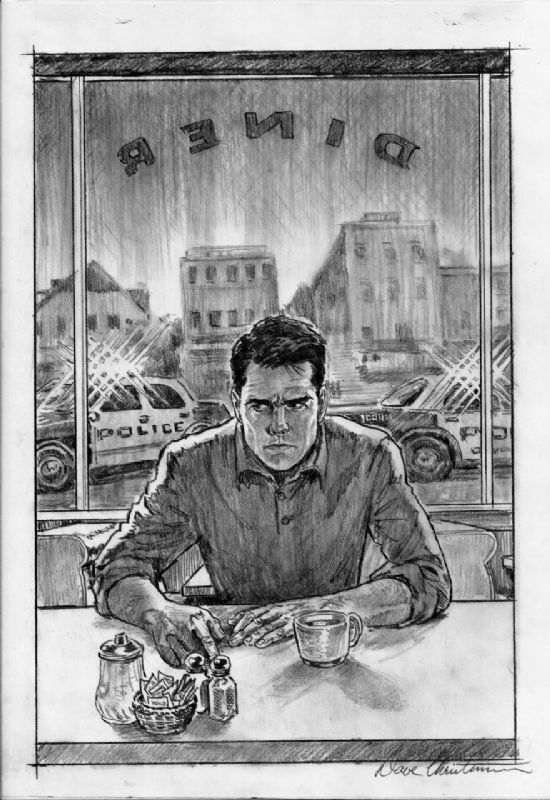This black and white pencil illustration appears to be a scene from a graphic novel or movie. It shows a distressed man with short, dark hair sitting at a counter in a diner, hunched over a cup of coffee. His formal long-sleeved shirt has its sleeves rolled up to the elbows. He is glancing suspiciously over his right shoulder, anxious not to let the police catch sight of him. Behind him, through clear windows, is the backward lettering of the word "diner." Beyond the glass, two police cars with flashing sirens are parked on either side, casting light onto the scene. In the background, typical city buildings line the street. On the counter in front of the man are salt and pepper shakers, a sugar dispenser, and a basket likely containing sweetener packets. The lower right corner of the image bears a cursive signature, partially readable as "Dave."